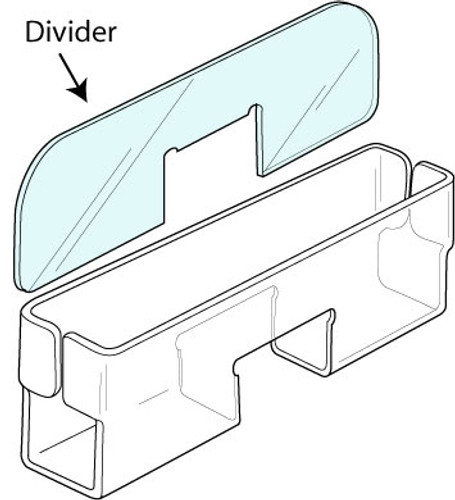The black and white image appears to be a detailed technical drawing, resembling an illustration from an instruction manual. It features a clear or potentially transparent rectangular container that has openings on its sides, top, and bottom. Inside this container is a thin, light-blue-hued piece labeled as a "divider" by an arrow and text in the top left corner of the image. The divider is designed to slide into or be placed inside the larger container, suggesting modular functionality. This configuration could indicate that the container and its divider are meant to stack or be organized in multiples, although the exact size and intended use remain unspecified. The simplistic, color-outlined design hints that the container and the divider could be fabricated from either plastic or metal, with no definite clues to the precise material or the specific application.